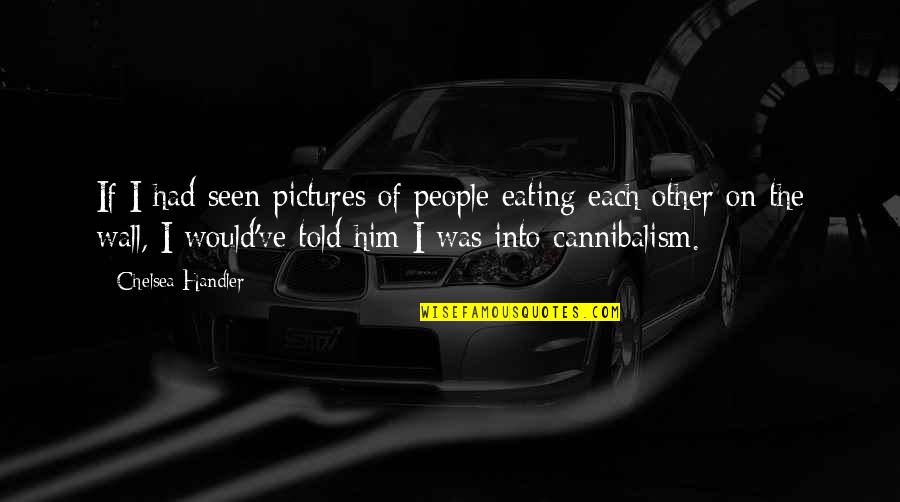This is a horizontal rectangular image with a black background that features faint gray lines, which might represent a street or other abstract design, allowing for some imagination. At the center of the image, there's a black and white, somewhat blurry photo of a car, which appears gray due to the black and white treatment. Behind and to the right of the car, there are two indistinct circles and a tunnel-like structure. 

Overlaying the middle of the image is a white, small-font text that reads: "If I had seen pictures of people eating each other on the wall, I would have told him I was into cannibalism." This quote, attributed to Chelsea Handler, is written in a somewhat Frankenstein-y font. Beneath this, in a typewriter-like font within a yellow rectangle, is the source "wisefamousquotes.com." The overall quality of the image is low, contributing to the difficulty in discerning some details.